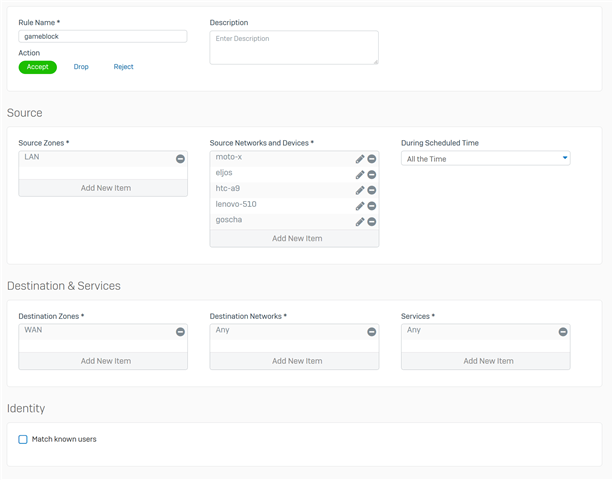The image depicts a router settings interface on a gray background with four distinct white sections for configuring network scheduling rules. At the top section, labeled "Rule Name" with an asterisk, a text block contains "Game Block". The "Action" field offers options: "Accept" (in a green button with white text), "Drop," and "Reject" (both in blue).

To the right, the "Description" field includes a text box prompting "Enter description". Below, the "Source" section begins with "Source Zones" marked by an asterisk and pre-filled with "LAN" alongside a gray delete icon. An "Add New Item" button is available. 

Next are "Source Networks and Devices" featuring entries such as Moto X, ILJOS, HTC A9, Lenovo 510, and Gosha, each with "Edit" and "Delete" buttons and an "Add New Item" option. The "During Schedule Time" setting is set to "All the time".

The "Destination Services" portion shows "Destination Zones" pre-filled with "WAN" and a delete option, and "Destination Networks" set to "Any" with a delete option. Similarly, "Services" is also set to "Any" with a delete option. Each category here offers an "Add New Item" button as well.

Lastly, the "Identity" section contains "Match Known Users" with a selectable blue box next to it.